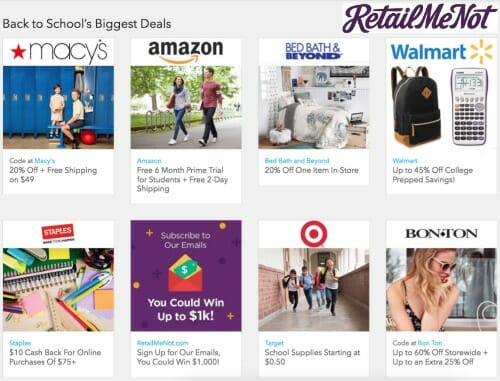In this screenshot featuring a website page set against a white background, the viewer's attention is drawn to a light lavender header at the top. The header prominently displays "Back to School's Biggest Deals" in dark gray text positioned on the upper left side. On the upper right, slightly cursive and bold text spells out "Retail Me Not."

Beneath the header, a series of advertisements from various stores are showcased. The first advertisement on the left is from Macy's, marked by their iconic red star logo. It features an image of two young kids standing in front of a locker room, holding a ball. The promotion beneath the image states, "20% off and free shipping on $49." 

Next is Amazon, which offers a "Free six-month prime trial for students and free two-day shipping." The accompanying image shows two students walking outside along a path. 

To the right is an advertisement for Bed Bath & Beyond, showcasing a cozy bedroom scene. 

Following that is Walmart's ad, which depicts a backpack on the left side and a calculator on the right, with "Walmart" written in blue text. 

On the lower left, Staples features school supplies in their advertisement. 

Lastly, Target and Bon-Ton round out the collection of deals, with their respective promotions and images included in the layout.